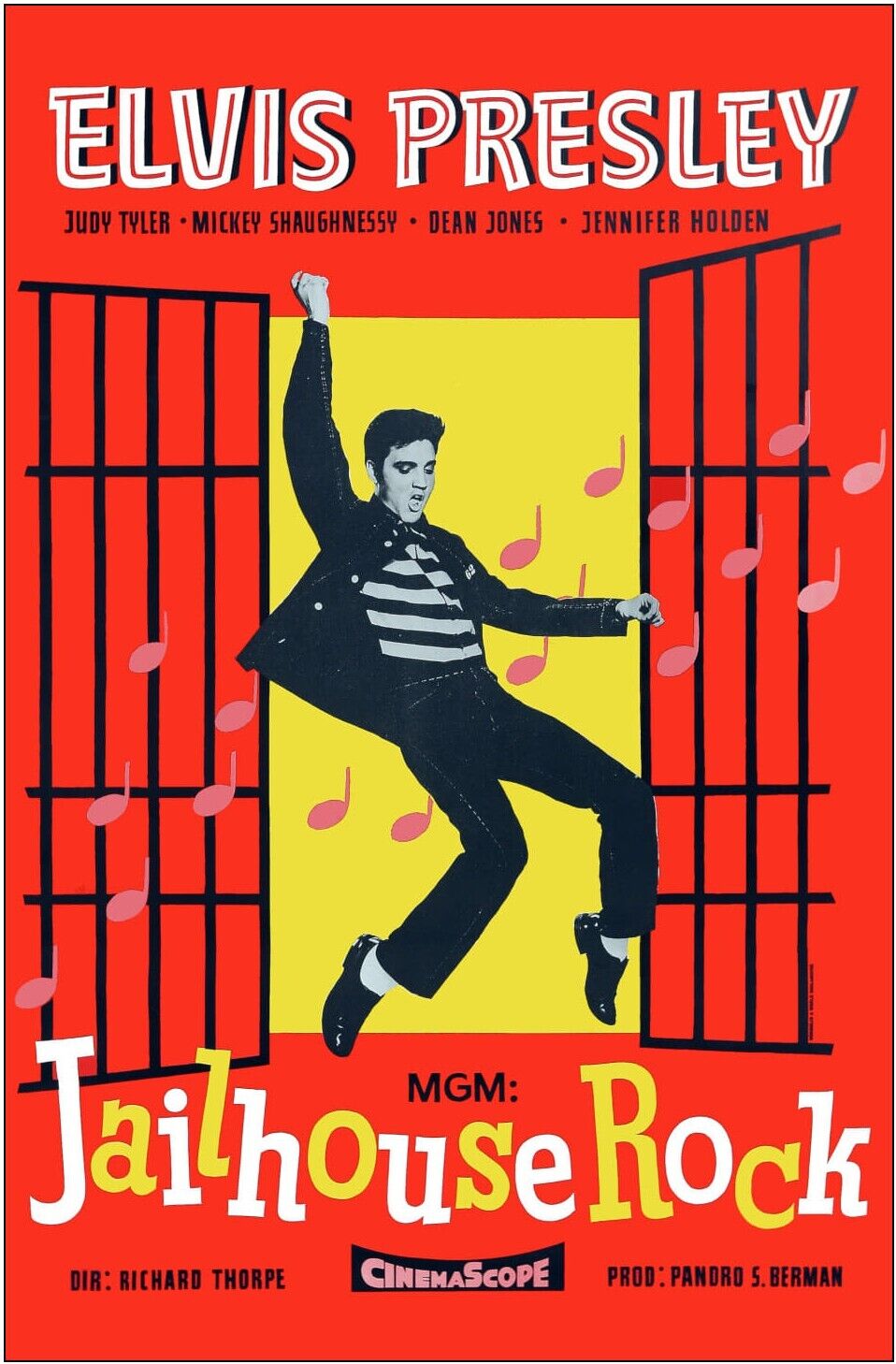This vibrant, full-color advertisement showcases the iconic movie "Jailhouse Rock" featuring Elvis Presley. Set against a striking bright orange-red backdrop, the central focus is a large yellow rectangle framing Elvis Presley himself. Elvis, captured mid-dance on his tiptoes in one of his famous moves, dons his iconic black-and-white striped prison t-shirt beneath a black jacket, paired with black slacks, white socks, and black shoes. Prominently displayed above him are his name in large letters and the names of co-stars Judy Tyler, Mickey Shaughnessy, Dean Jones, and Jennifer Holden. The jail bars flanking him are adorned with pink musical notes, adding a whimsical touch to the scene. The poster credits MGM, mentions the director Richard Thorpe, and highlights that the movie was produced by Pandro S. Berman and shot in CinemaScope.